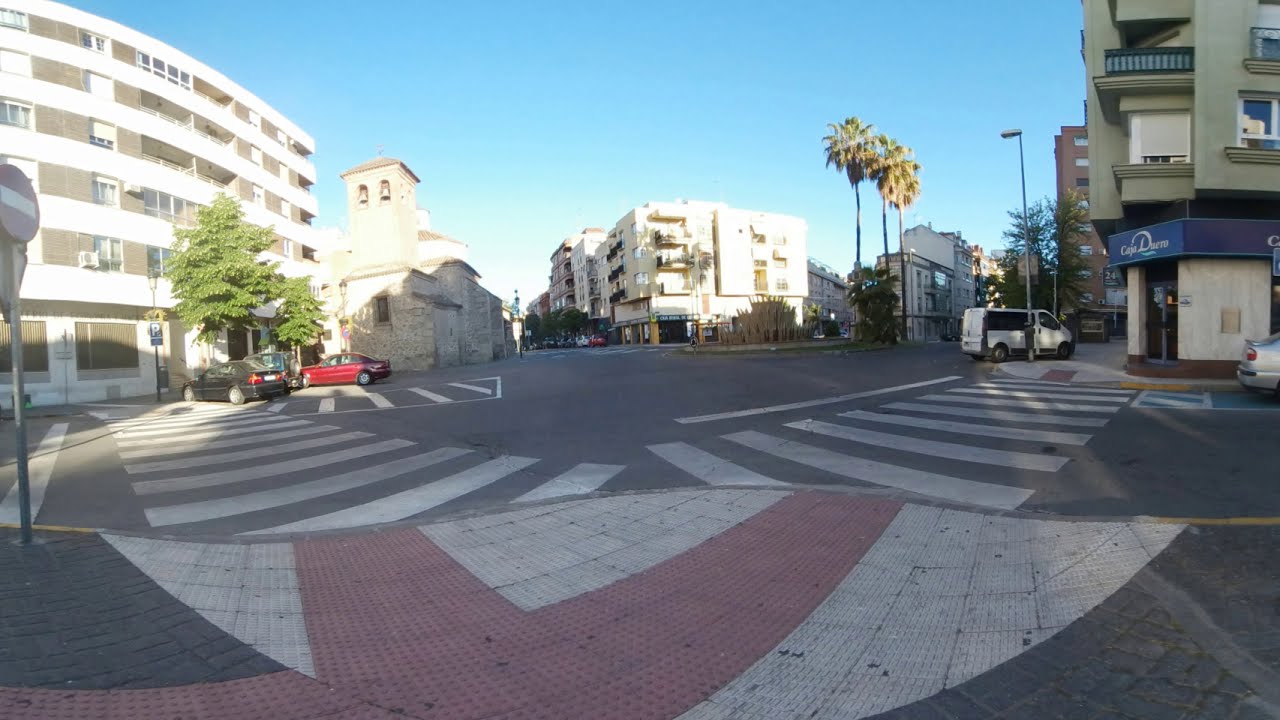This photograph captures a vibrant city street scene in a likely southern hemisphere city. Central to the image are two white-striped crosswalks that extend from the center to both the left and right sides of the frame, defining a bustling intersection on a grey concrete street. The background showcases an array of buildings with varied architectural designs and hues, predominantly in white and tan, with several displaying numerous windows and balconies.

On the left side, a six-story white building with balconies is prominent, while on the right, an olive-colored building with a café and a blue awning at its base adds color to the scene. The street below is dotted with several parked vehicles: a white minivan, a red car, and a black car, both of the latter appearing to be BMWs. Additionally, a darker-hued vehicle, possibly a jeep, is noticeable amidst the line of parked cars.

Palm trees frame the sidewalk, providing a distinct tropical touch, with several tall specimens rising above the buildings. The sky overhead is a clear, cloudless blue, enhancing the bright and lively ambiance of the cityscape. Overall, the view down this main street blends urban architecture and nature seamlessly, offering a picturesque snapshot of urban life.